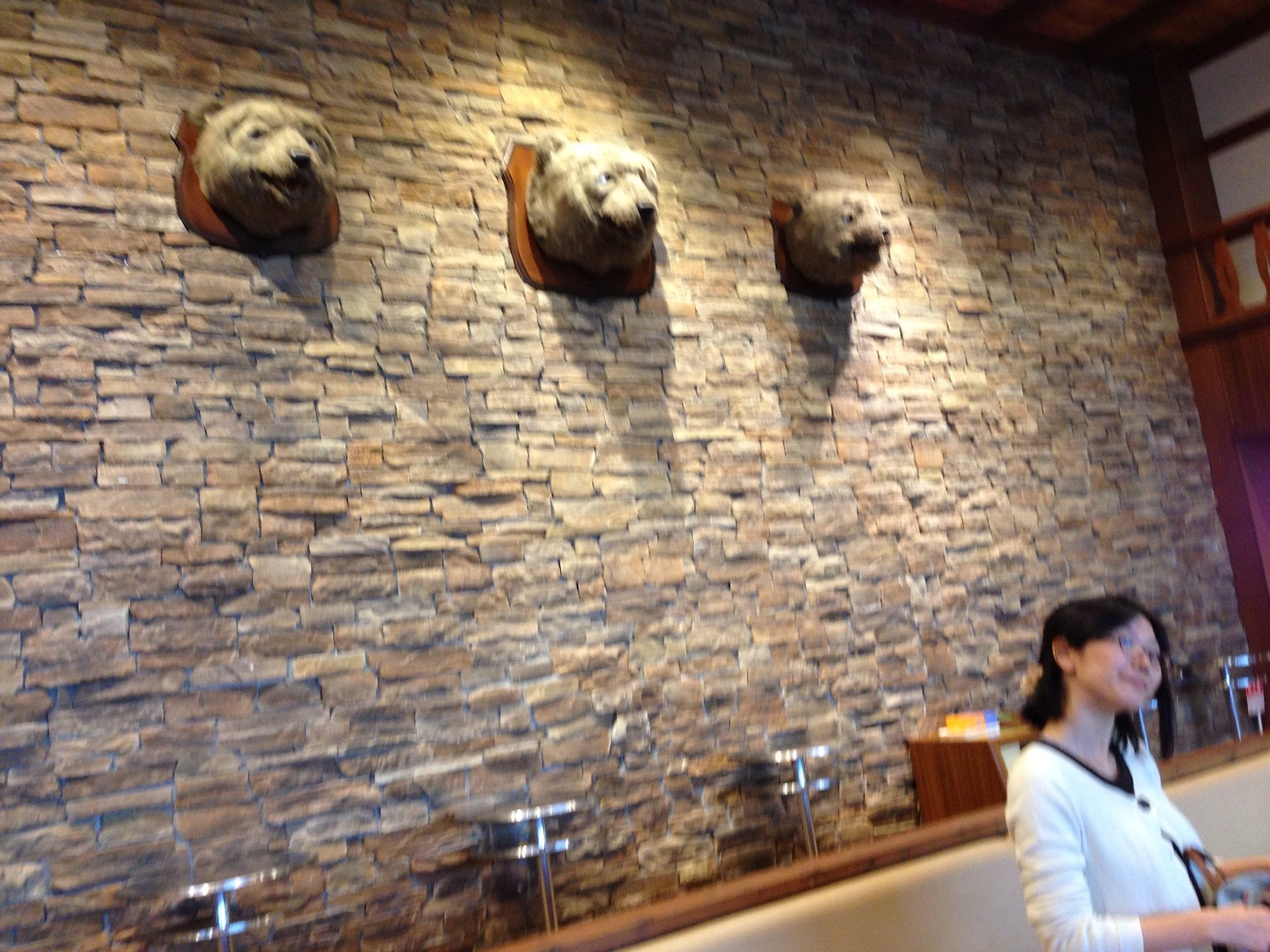The image depicts the interior of a restaurant with a rustic and trophy-themed décor. Dominating the scene is a large wall constructed from various shades of brown and off-white stone, adorned with three mounted bear heads arranged like trophies. Each bear head appears to be spotlit, though one is somewhat dimmer than the others. Against this striking backdrop, there are three identical metal structures, possibly trays or fixtures, aligned at the back.

In the lower right portion of the image stands a woman, who may be the restaurant's hostess or a customer. She has dark hair, wears glasses, and is dressed in a white blazer over what appears to be a black shirt. Her interaction seems poised and attentive, though only her upper body is visible. The ceiling above features wooden beams that add to the rustic ambiance. Directly behind the woman is a light-colored surface, potentially a table or a bar counter, adding contrast to the darker elements in the scene. Overall, the setting exudes a warm yet somewhat eerie atmosphere, highlighted by the taxidermied bear heads.